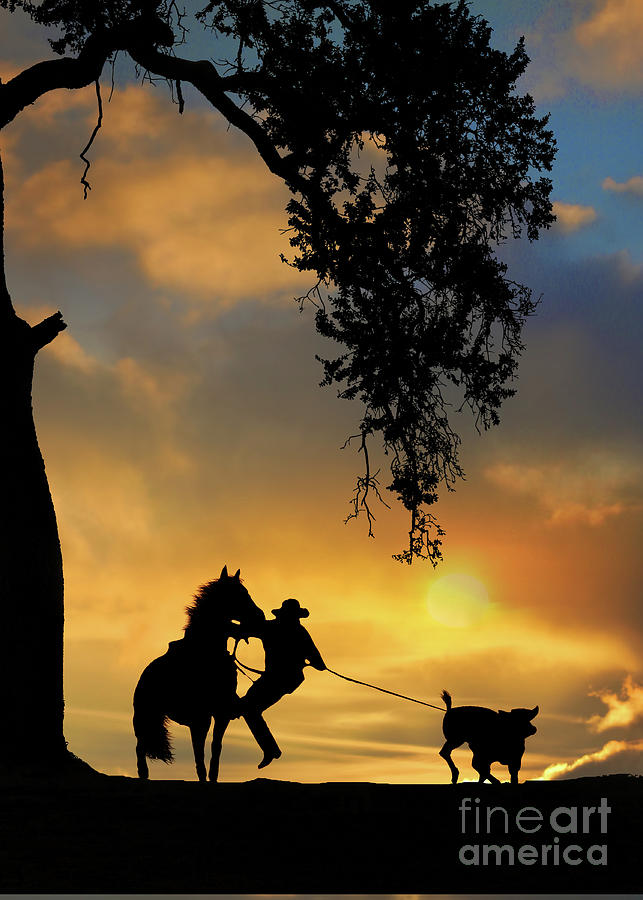The image is a professional fine art photograph captured at sunset, showcasing a dramatic silhouette against a vividly colorful sky of blues, reds, and oranges. In the foreground, a cowboy, distinguishable by his hat, is seen either getting on or off his horse. The cowboy holds a rope that is attached to an animal, most likely a bull or a pig, in his other hand. Both the cowboy, the horse, and the animal are rendered in striking black silhouette. To the left, a tall tree with a prominent branch drooping down frames the scene, adding depth and context. The bottom portion of the image is solid black, representing the ground. The text 'Fine Art America' is subtly placed in the lower right corner, marking the artistry and authenticity of the photograph. The ambient light from the setting sun peeks through the clouds, casting a vivid yet serene glow over the entire composition, evoking a sense of timeless western Americana.